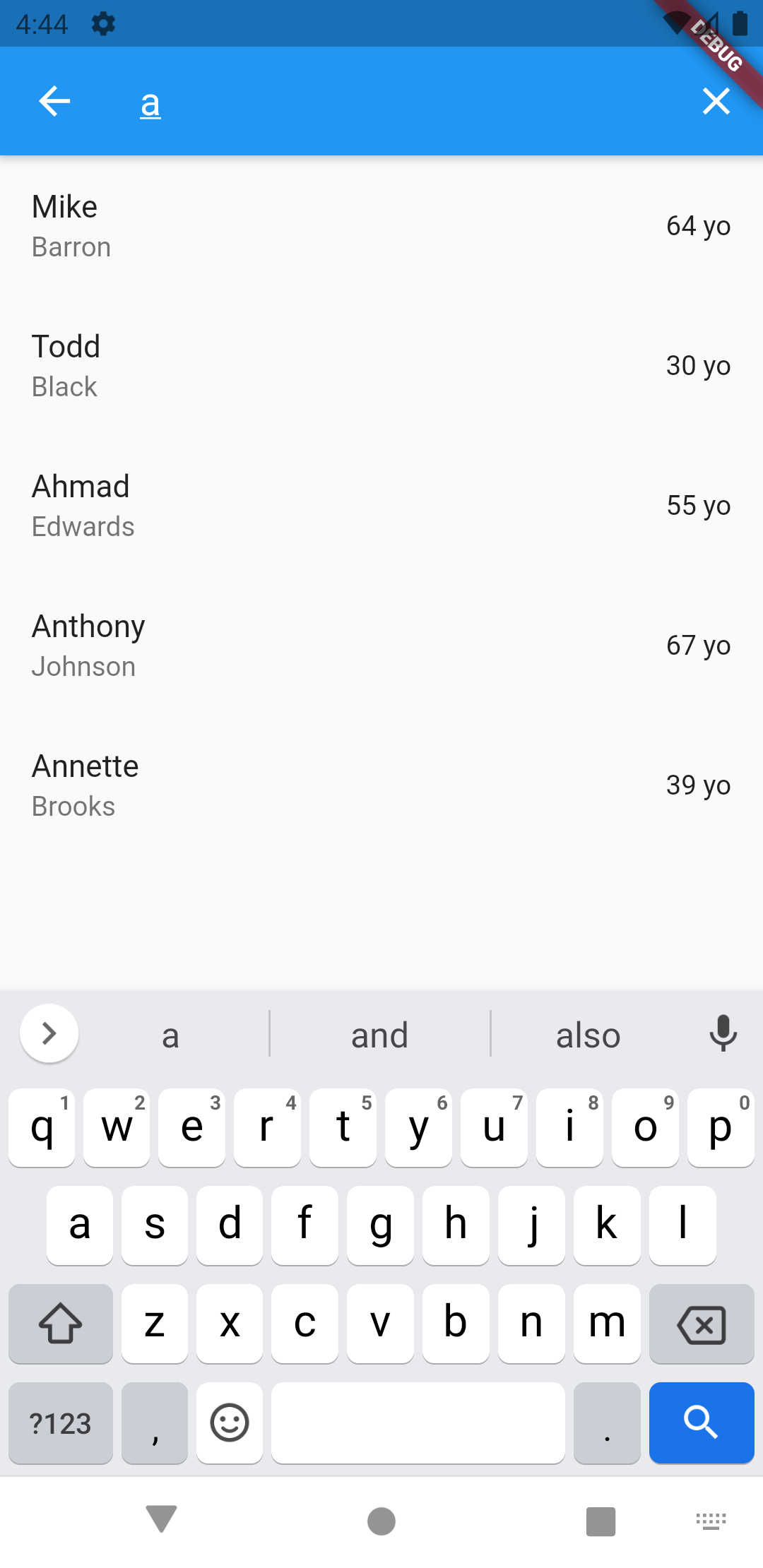The image is a screenshot captured from a mobile device. At the very top, there's a thin dark blue banner stretching across the screen. In the left corner of this banner, the time is displayed as 4:44, accompanied by a flower icon. To the right, there are icons indicating cellular signal strength, Wi-Fi signal, and battery life. A small red banner in the top-right corner features the word "debug" in white lettering.

Beneath this, there's a slightly thicker and lighter blue bar. On the left side of this bar, there's a white back arrow followed by the letter 'A' also in white. On the right side of this bar, there's an 'X' or close button.

Below this bar, a list of names and ages is presented: Mike Barron, 64; Todd Black, 30; Ahmaud Edwards, 55; Anthony Johnson, 67; and Annette Brooks, 39. At the bottom of the screen, the mobile device's keyboard is visible, suggesting that text input is active.